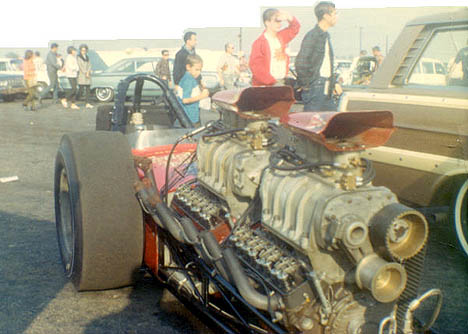This photograph exudes a vintage ambiance, likely capturing a moment in a parking lot or at a historical event. Dominating the foreground are two powerful engines, potentially V6 or V8 models, prominently mounted at the front of the showcased vehicle. On the vehicle's left side is a visible tire, with the rear right tire being notably large and thick, reminiscent of a Formula 1 tire. The exposed parts of the vehicle are painted in bold red, highlighting its open-engine design.

In the top right quarter of the image, the back of a station wagon is discernible, indicative of the era's automotive style. The background reveals a bustling scene with several people walking from left to right, their attire reflecting the fashion of the 70s or 80s. The array of vintage cars further situates the image in an older period, creating a nostalgic snapshot of a bygone era.